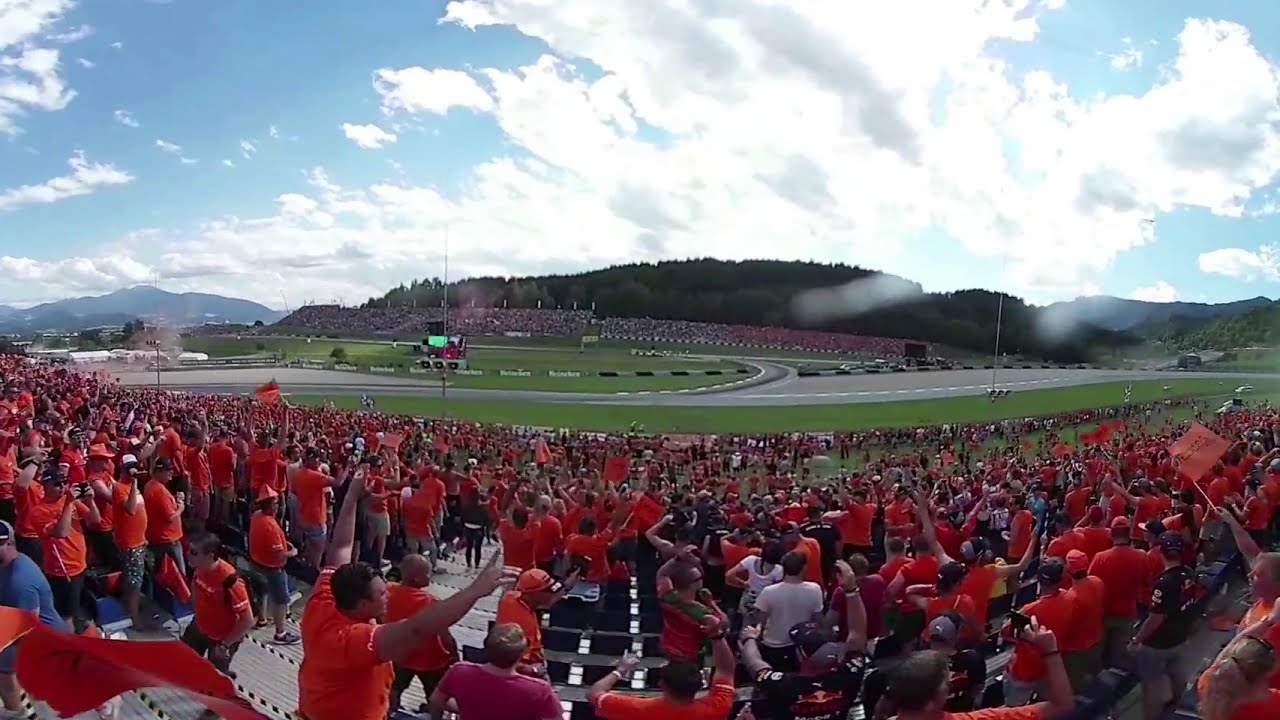This photograph captures an exciting car race event, possibly a NASCAR race, set in an expansive outdoor speedway surrounded by low rising hills covered in trees. The clear blue sky is dotted with fluffy white clouds, framing the scene. In the foreground, large crowds fill the bleachers, all enthusiastically clad in matching red or orange-red t-shirts, waving flags of the same color, clearly supporting their favorite teams. The bleachers descend in steps toward the manicured grass area below, which features curved intersecting roadways, possibly part of the racetrack's design. Distant stands on the far side of the grassy area are also filled with spectators, highlighting the grand scale of the event. The photo, taken from behind the stands, gives a panoramic view of the racetrack, where cars speed by on the asphalt track, encapsulating the high-energy atmosphere of the race.